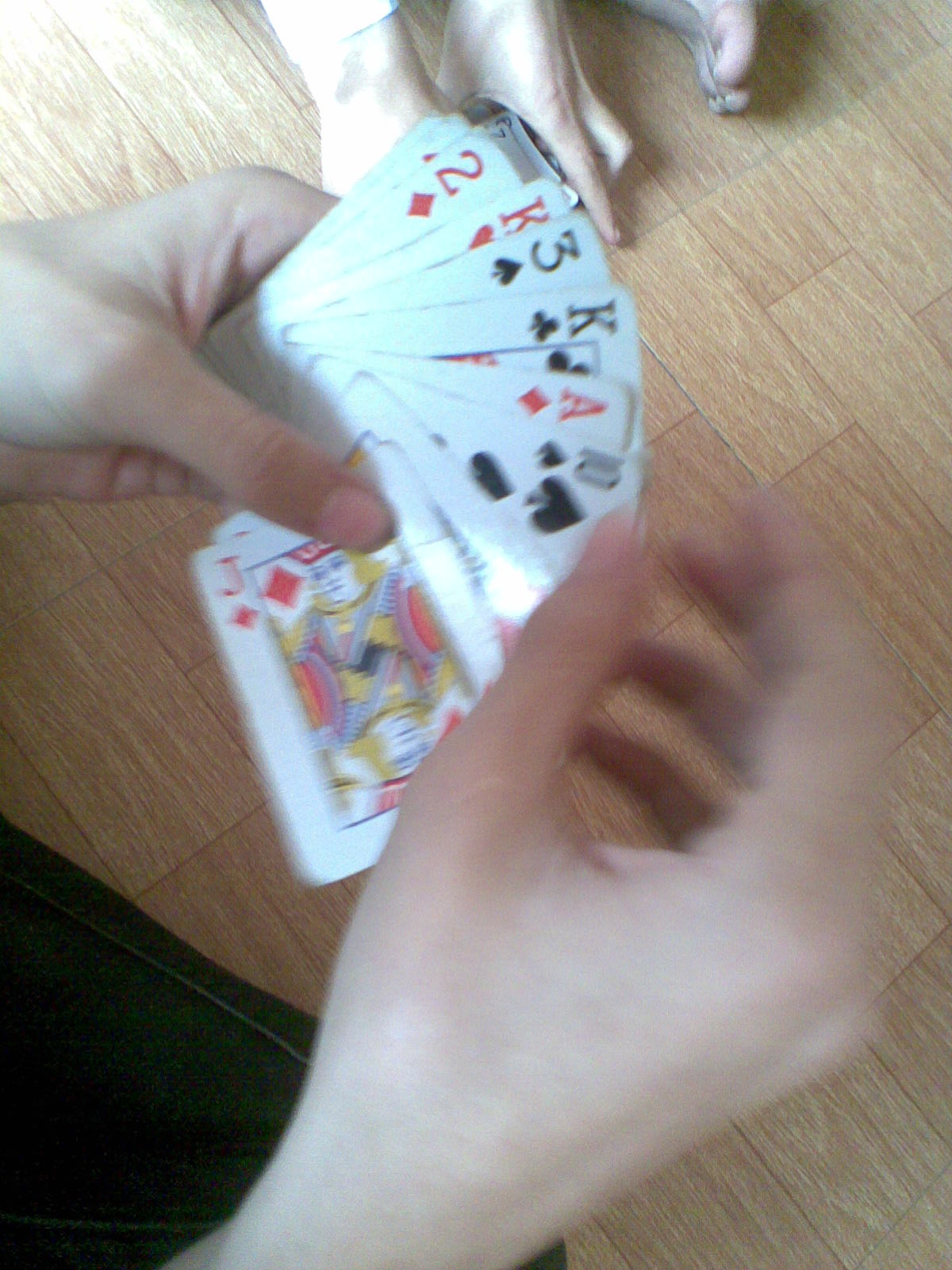This is a detailed portrait-style image taken with a camera, focusing on a white hand emerging from the middle bottom of the frame. A second white left hand enters the frame from the top left corner, holding a fan of approximately ten playing cards. Each card is meticulously positioned to display its number. The sequence from left to right includes the two of diamonds (red), king of hearts (red), three of spades (black), king of clubs (black), ace of diamonds (red), and ten of spades (black). The next card is obscured by the thumb, followed by the partially visible bottom of the jack of diamonds. The background comprises a light brown hardwood-tiled floor. At the top of the image, a person's toes are visible, along with both hands— the right one beneath the cards and the left with the webbed space between the index finger and thumb peeking out around the two of diamonds.